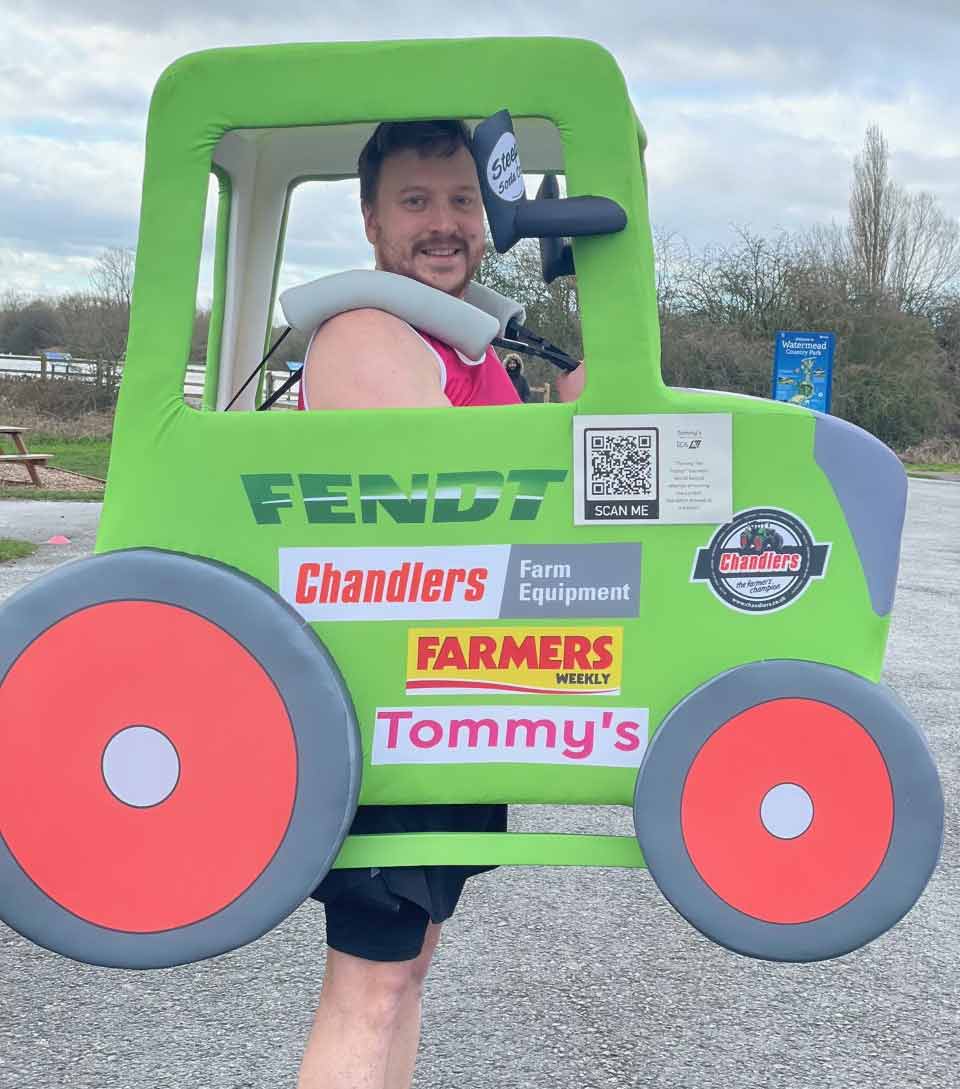In this lively and humorous photo taken in a parking lot, an adult man is posing and smiling cheerfully while wearing an eye-catching costume resembling a green farm vehicle with black tires and red rims. The costume has padded shoulder supports, allowing it to be worn over his shoulders. The man's face is clearly visible through the open window spaces of the vehicle. He is dressed in a bright fuchsia tank top and black shorts, adding to the vibrant appearance. His costume is adorned with several logos, including "FENDT," "Chandler's Farm Equipment," "Farmers Weekly," and "Tommy's," all promoting various businesses. Furthermore, there is a QR code labeled "scan me," providing onlookers a way to easily access more information. The man, who has a beard and mustache, appears to be thoroughly enjoying himself.